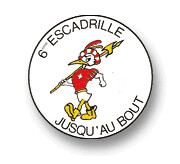The image depicts a round pin featuring a cartoon bird, which appears to be a duck with yellow legs and a pointed beak. The duck is marching with a serious expression, holding a halberd—a staff with a flat blade. Dressed in a red short-sleeved shirt adorned with a white cross, the duck also wears a red and white striped hat with two feathers on top. Additionally, the duck is clad in yellow work boots. Text encircles the image: "6-ESCADRILLE" at the top and "JUSQU'AU BOUT" at the bottom. The entire scene is framed within the circular pin, a likely accessory for wear on a hat or lapel.